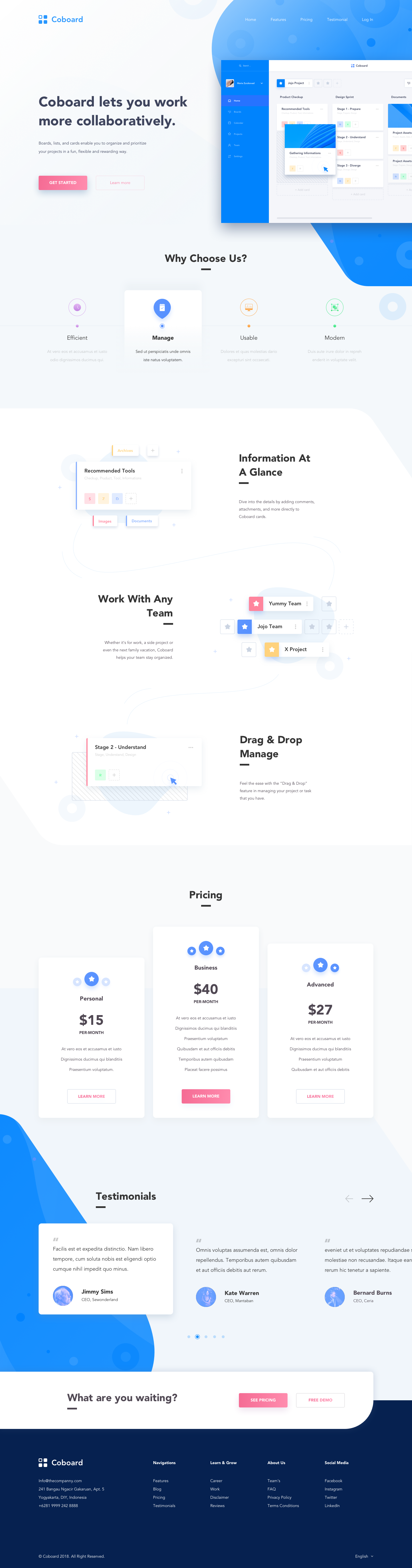**Caption:**

A comprehensive screenshot of the Coboard webpage showcases its collaborative work tool designed for team project management. Coboard emphasizes enhancing teamwork with features such as boards, lists, and cards that allow users to organize and prioritize tasks in a fun, flexible, and rewarding manner. Prominently displayed are options to get started or learn more about the tool. The page highlights the advantages of choosing Coboard, citing its efficiency, managed workflow, usability, and modern design. 

The image further emphasizes the functionality of presenting information at a glance and recommends tools for more detailed project management. Users can add comments and attachments directly to Coboard cards. It demonstrates compatibility with various teams, listing examples such as Yummy Team, Jojo Team, and X Project. The intuitive drag-and-drop feature is illustrated with stages of project management, emphasizing the ease of use.

Additionally, the pricing section outlines the cost: $15 per month for personal use, $44 per month for business, and $27 per month for advanced features. The screenshot concludes with customer testimonials and a call to action, encouraging potential users to see the pricing details and explore how Coboard can benefit their workflow. The webpage ends with the Coboard logo and contact information, completing a thorough overview of its offerings.